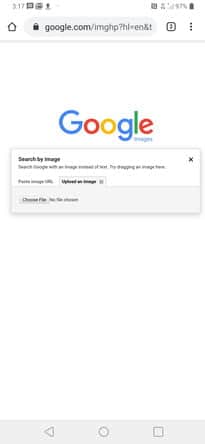The image appears to be a screenshot from a phone. The screen displays a web browser interface with various elements in different states of clarity.

In the top-left corner, there is a faded time display reading "3:17," with a few square blackish icons next to it. On the top-right, a battery icon indicates 97% battery power.

Below, on the left side, there is a black outline of a house icon. Further down, a gray-outlined circle containing a black padlock is present. Inside the circle, there's a faded text in black font reading "google.com/IMGHP," followed by a light gray font with the text "?NL=EN!" next to a black box and three vertical dots. A gray line extends underneath this section.

The Google logo appears prominently in the middle of a white background with each letter colored respectively: the G in blue, the first O in red, the second O in yellow, the second G in blue, the L in green, and the E in red. Underneath the logo, the word "Images" is written in blue just below the final "E."

Below the Google logo, there is a black-font text reading "Search by image" to the left of a small "X" icon. Some very faint light gray text follows to the right of this.

Further down, more text appears in a combination of gray and black fonts. Black text under a gray square is noticeable, followed by another section with very faded gray wording on a light gray background. 

At the very bottom, after a considerable white space, there is a gray box featuring multimedia control icons: a triangle pointing left (representing play/pause), a circle in the middle, and a square to the right, all displayed in gray font.

The entire image seems to be a standard interface of a search engine, specifically Google's image search page, captured on a smartphone.